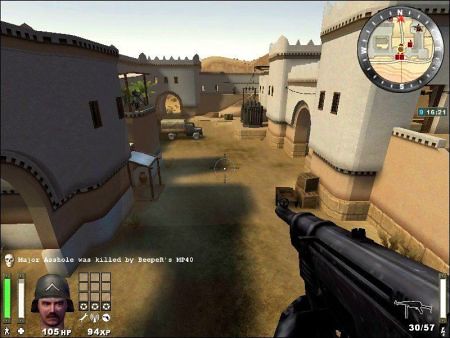The frame captures a horizontally rectangular screenshot from a video game, featuring an immersive and detailed scene. Prominently displayed in the lower right corner is the end of a black, rifled barrel, directed towards the center of the screenshot. The backdrop showcases tall, castle-like buildings that contribute to an imposing medieval ambiance. These structures exhibit a gradient color scheme, with tan hues at the base transitioning to light gray as they ascend upwards.

In the upper right corner of the image, a detailed compass is visible, providing crucial in-game navigation. Inside the compass, there is a miniature map of the area, pinpointing the exact position of the rifled barrel, thereby orienting the player within the environment. Additionally, the lower right corner features an overlay display that includes various statistical information—presumably health, ammunition, and other relevant game metrics—alongside the player’s avatar or image, enhancing the strategic elements of gameplay.

Overall, the screenshot vividly captures the essence of the game's interface and setting, blending atmospheric architecture with essential gameplay mechanics in a complex and visually coherent manner.